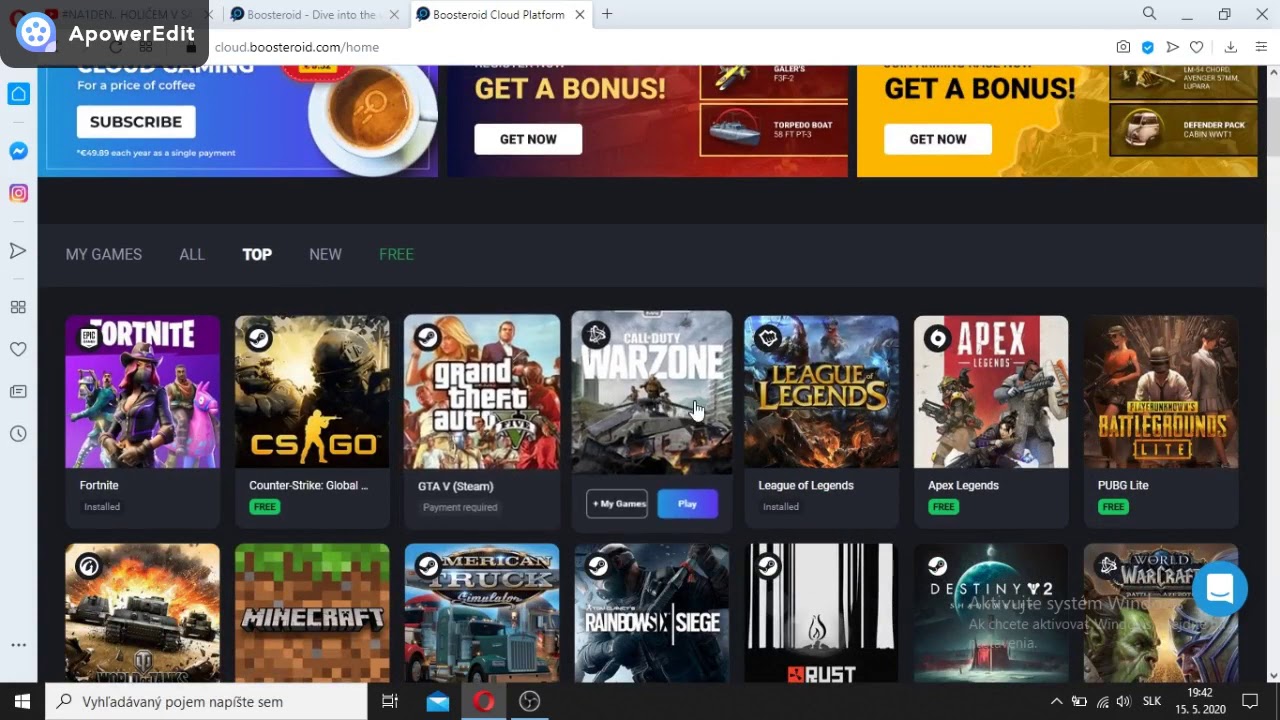The screenshot captures the homepage of a website displayed on a desktop computer. The browser address bar at the top reveals the URL: "cloud.boosteroid.com/home," located adjacent to a gray rectangular icon. Below the address bar is the homepage, which features a vibrant and colorful layout against a black background. The main content of the page highlights an assortment of games arranged in two horizontal rows, each row containing seven game covers, making a total of 14 games displayed. In the upper row, the first game featured is "Fortnite," characterized by its distinctive purple cover art. Adjacent to it is "CS:GO," recognized by the outline of a soldier holding a gun, creatively integrated between the letters 'S' and 'G.'